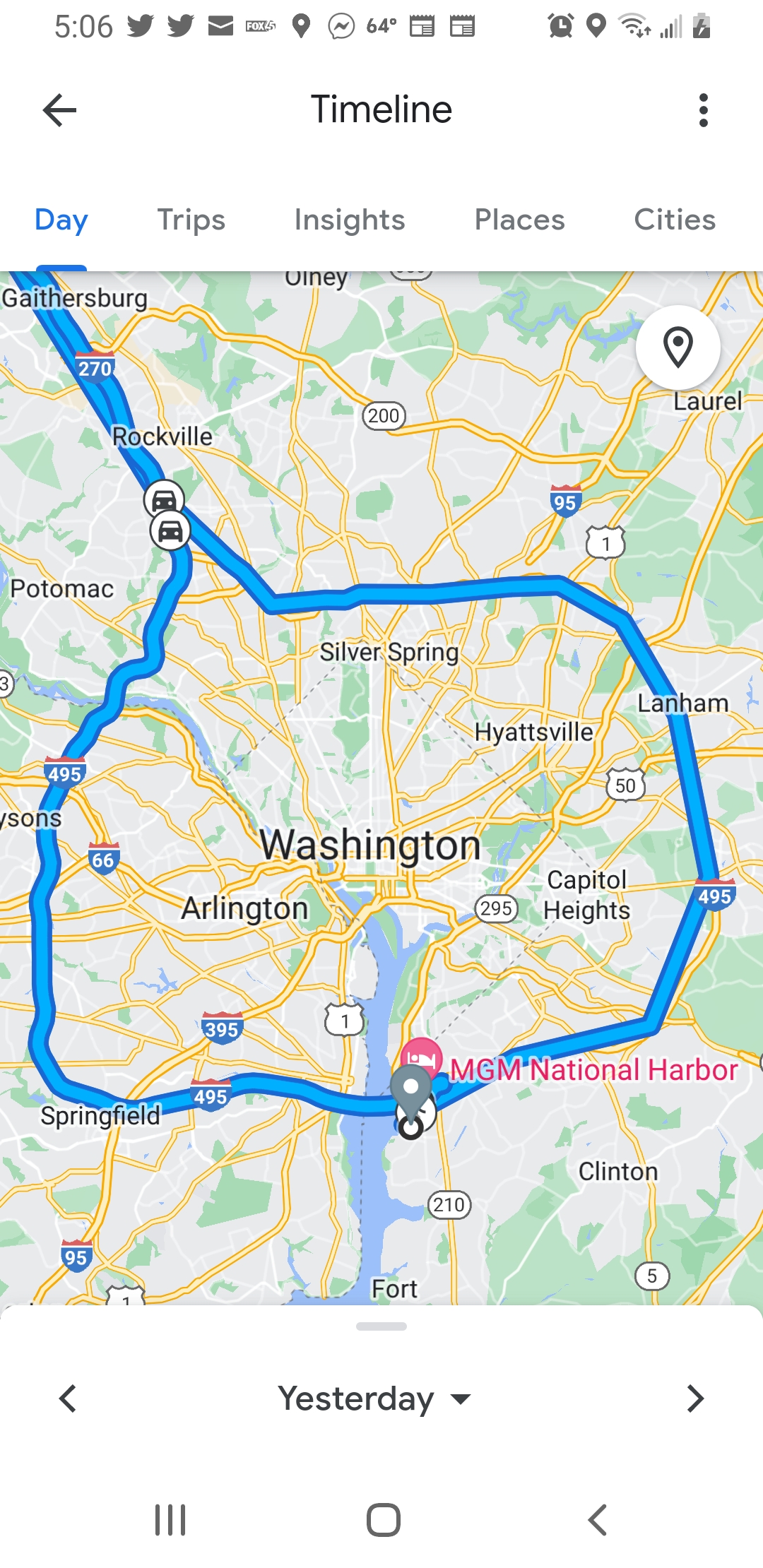A screenshot of a smartphone map interface is displayed, indicating it was captured on a mobile device due to the visible status bar at the top, which shows icons for Twitter, email, the current temperature, and an alarm. Underneath the status bar, the interface shows menu options labeled "Timeline," "Day," "Trips," "Insights," "Places," and "Cities." The map itself prominently features a large blue circle centered around Washington, DC, with a route extending towards the upper right corner, leading into Maryland. This suggests that the map is displaying directions for a route originating in Maryland and heading towards a destination in Washington, DC.